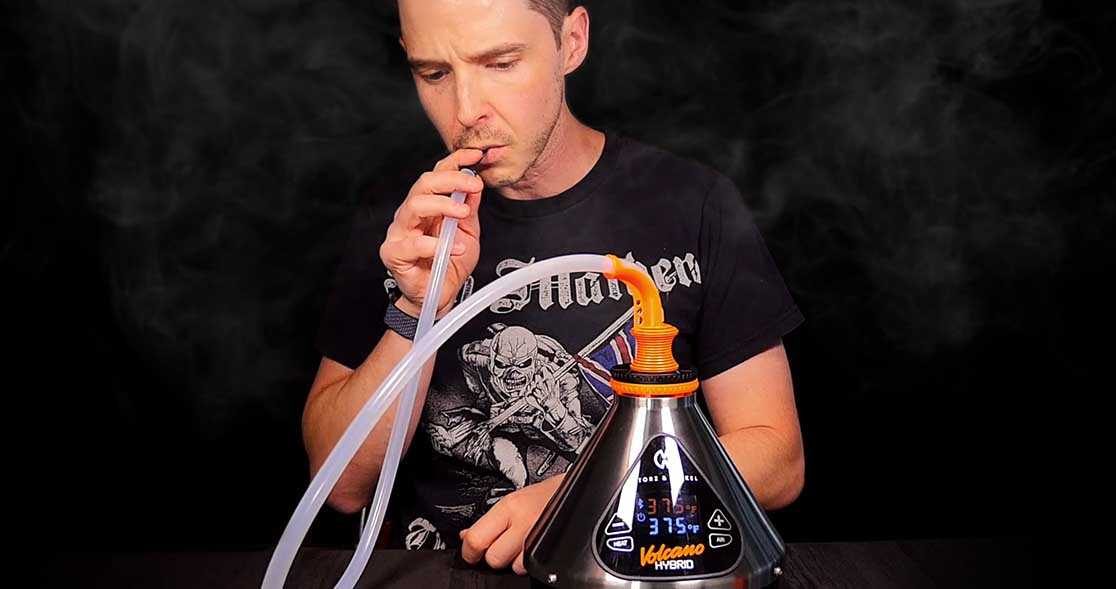The image is a rectangular photograph capturing a man from his waist upwards, set against a solid black background with wisps of thin smoke surrounding him. The man, who has short brown hair and a slight mustache, is dressed in a black T-shirt featuring a skeleton monster and the British flag, with "Van Halen" written above in white text. His right hand, adorned with a black wristwatch, holds a long white tube filled with smoke, which he's inhaling from. This tube is connected to a flask-shaped metal vaporizer called a "Volcano Hybrid," recognized by its orange top and LED screen. The vaporizer is specifically designed for cannabis or other herbs to ensure a cleaner inhalation experience. The man's left arm rests on his lap, visible just enough to complete the scene.